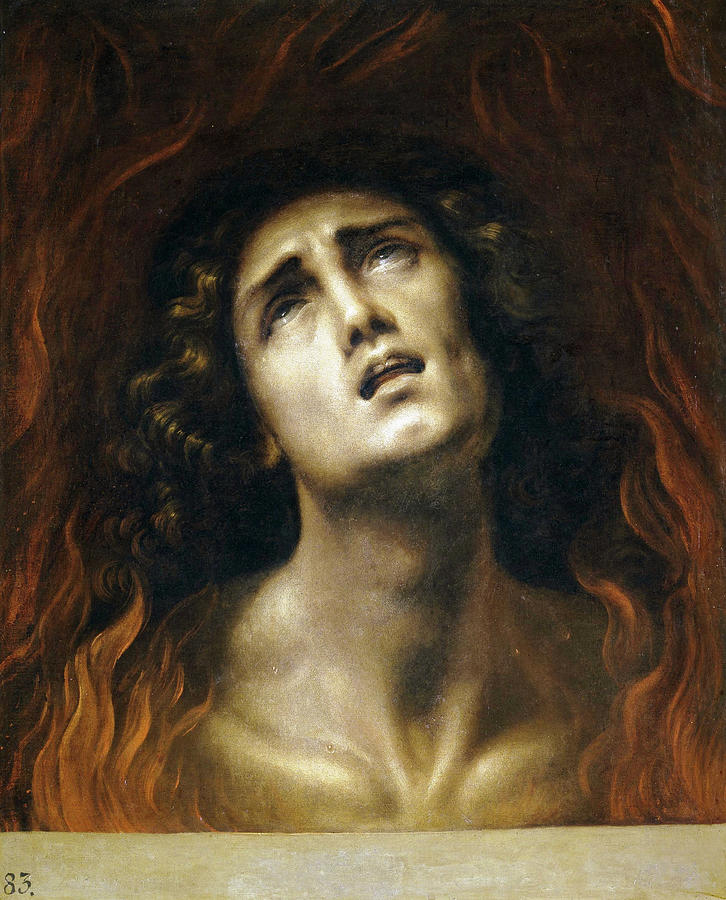The painting depicts a woman in profound anguish, captured from just above the breast upwards. She appears naked and is engulfed in golden-orange flames that ascend around her shoulders and the sides of her head, contrasting sharply with the black background. She is looking up to the sky, with her mouth open, revealing her teeth, and her eyes filled with tears that suggest immense suffering. Her brown hair flows to the sides, and she exhibits a clean-shaven face. In the bottom left corner of the painting, the number '83' is visible. It appears she might be standing next to a ledge or table.